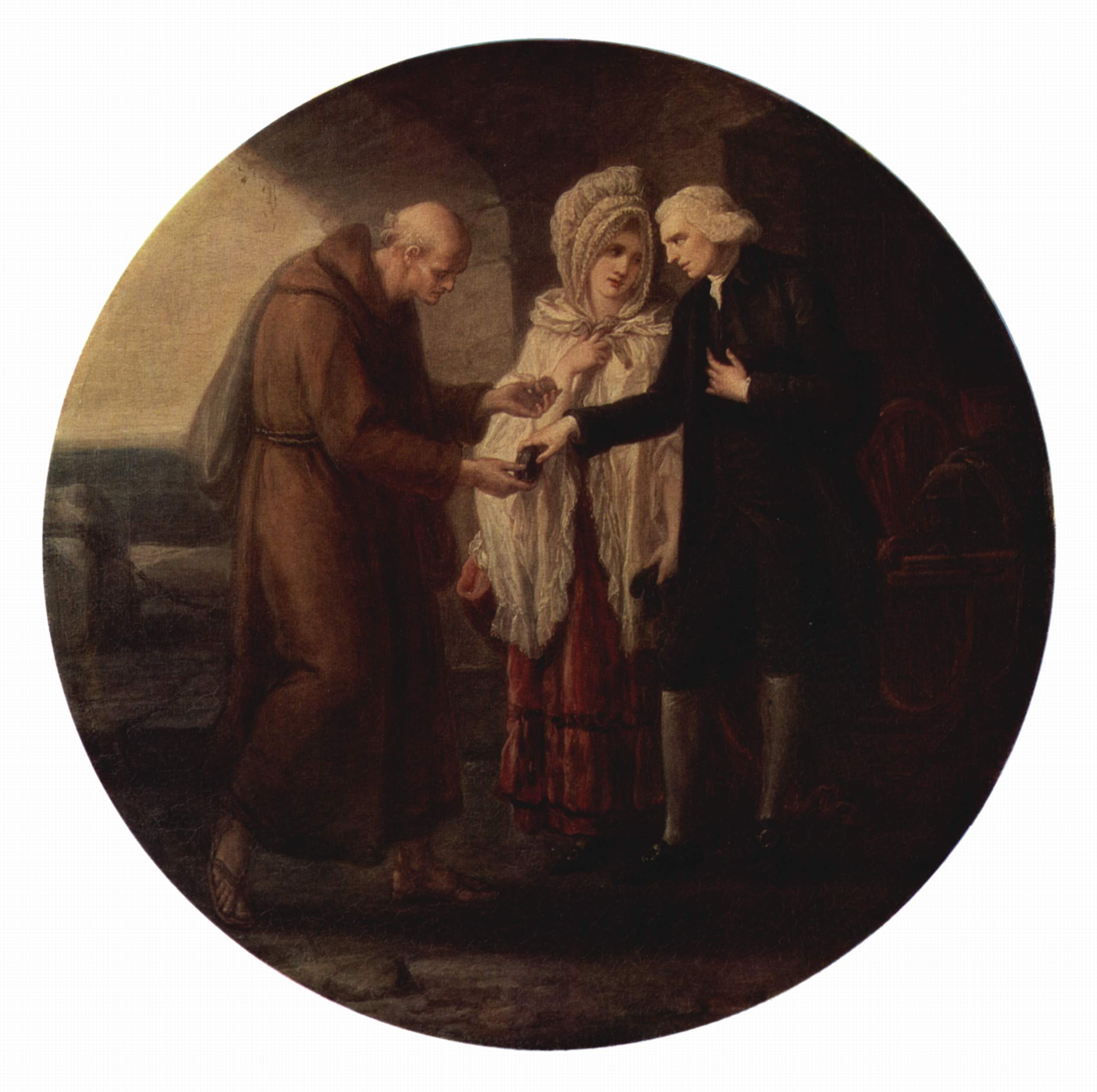In this detailed painting, framed within a perfect circle, a man and a woman appear to be engaging in an exchange with a friar or possibly a poor elderly man. The man, positioned to the right, is adorned in a colonial-style black suit reminiscent of the attire worn by prominent figures like George Washington or Thomas Jefferson. His outfit includes black shoes with gold buckles, white socks extending above his knees, and knee-length pants. His hair is white and wispy, contributing to his distinguished appearance. 

Standing closely beside him, a concerned woman in a white and red dress with a bonnet watches the interaction. The focal point of the scene is the man in the coat handing over a black bag, possibly filled with alms or goods, to the elderly bald man dressed in a simple brown robe and sandals. The setting is rendered in somber, dark, and earthy tones that evoke a twilight atmosphere, reinforcing the painting's historical and somewhat melancholic mood.